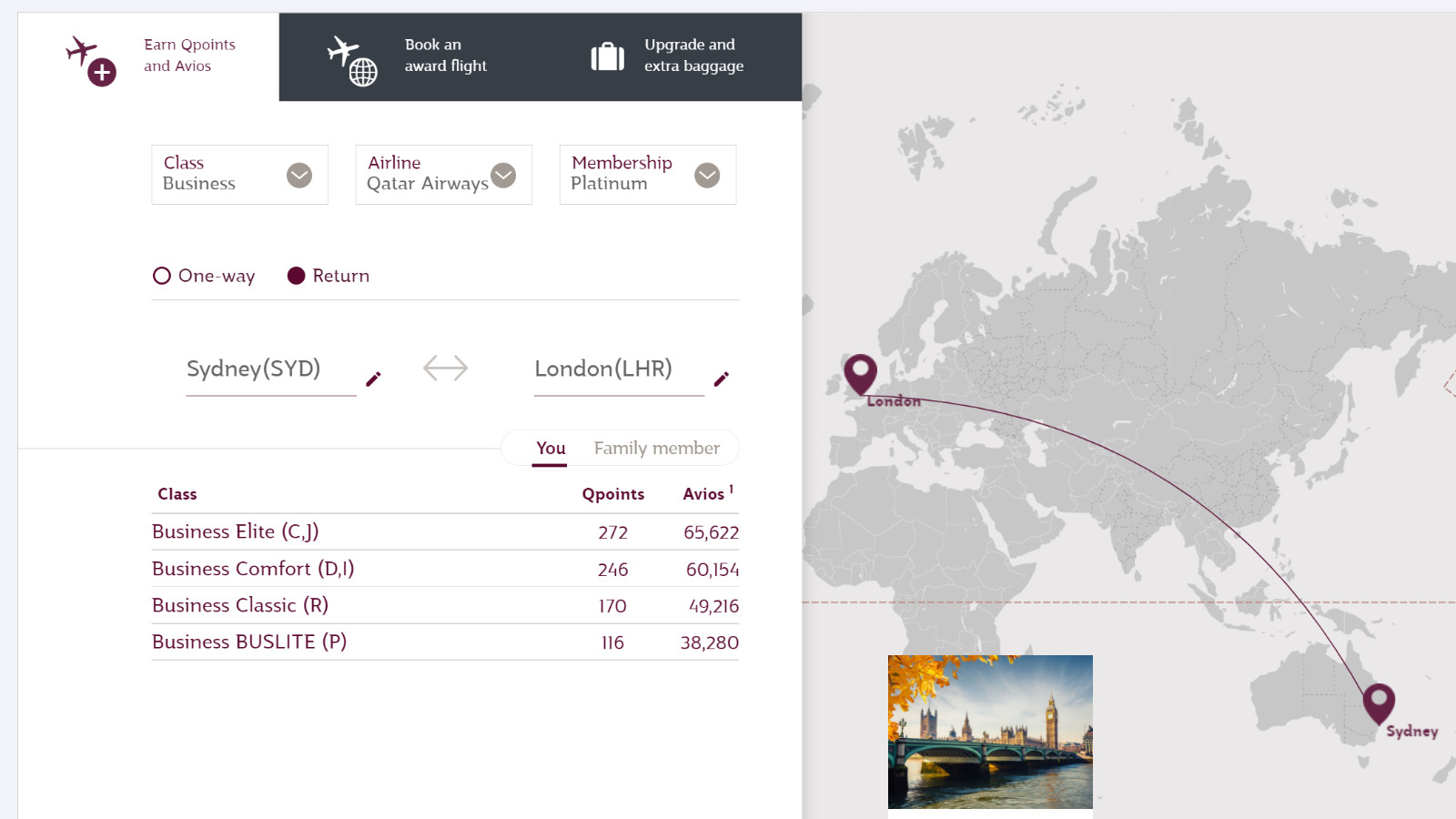This image features an interface reflecting a website or mobile app, presented in a rectangular layout approximately 1.5 to 2 times wider than it is tall. The layout is divided into two sections, with the left section occupying a bit over half of the space and the right section slightly under half.

The left side of the interface showcases three tabs at the top. The first tab, highlighted in white with a red overlay on its text, reads "Earn Qpoints and Avios" and includes an airplane icon with a plus symbol on its left. The other two tabs are shown with a black background overlay.

Beneath the tabs are three interactive buttons. Each button has its primary word colored in red, while the subsequent text is in gray. The buttons are labeled as follows:
1. "Class: Business" featuring a drop-down arrow.
2. "Airline: Qatar Airways" with a drop-down arrow.
3. "Membership: Platinum" with a drop-down arrow.

Further down, there is a selection for travel type, presented as radio buttons. The options are "One Way" (with an empty circle to the left, indicating it is not selected) and "Return" (with a filled circle to the left, indicating it is selected).

Below the selection options, there is a travel route displayed:
- On the left, "Sydney (SYD)" is indicated, followed by an editable field marked by a line beneath and a pencil icon to its right.
- An arrow pointing left and right separates the two locations.
- On the right, "London" is displayed with a similar editable field beneath and a pencil icon to its right.

This detailed depiction suggests an interface designed for booking flights, highlighting key features and user options.